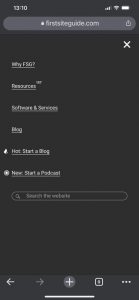This screenshot shows a very blurry and pixelated image of a phone screen displaying a web browser, likely Google Chrome in dark mode. The URL bar partially reveals the address, which appears to start with "firstsomethingguide.com," possibly indicating a site like "First Site Guide." 

Despite the low resolution, the site’s navigation links are somewhat discernible, including sections labeled "YFSG Resources," "Software and Services," and "Blog." Notable links include "Start a Blog" marked with "hot" and "Start a Podcast" marked with "new." The general appearance suggests a basic, instructional site focused on technology and entrepreneurial topics.

The screenshot also displays the browser interface, showing about eight or nine open tabs. Standard browser controls are visible, including options to exit the screen, add a new tab, and navigate back and forward. The dark mode theme along with the grainy quality of the image makes the text challenging to read, but the overall layout and function remain clear.